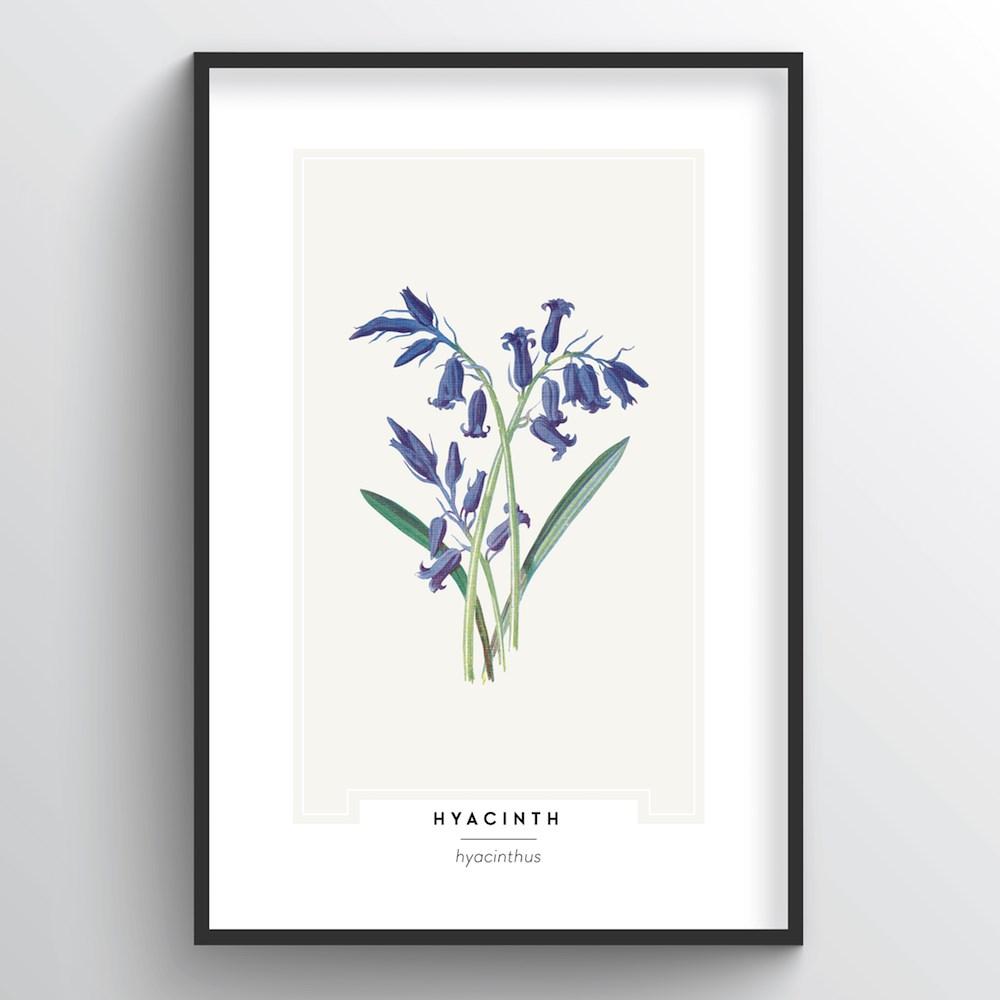A minimalist black-framed art print hangs on a white wall, illuminated by ambient light, giving the scene a subtle brightness. The vertically oriented frame encases a white mat that surrounds an off-white background, which showcases a striking botanical illustration. The central focus is a hyacinth plant, depicted in full bloom with vibrant purple flowers. Some blossoms stand tall, while others lie gently at their sides, revealing green stems and a green leaf on each side. Beneath the illustration, the text "HYACINTH" appears in bold, all-capital letters, with "Hyacinthus" written in lower-case italics beneath it, detailing the flower's scientific name. The art print exudes a clean, modern aesthetic, ideal for a contemporary kitchen or living space.